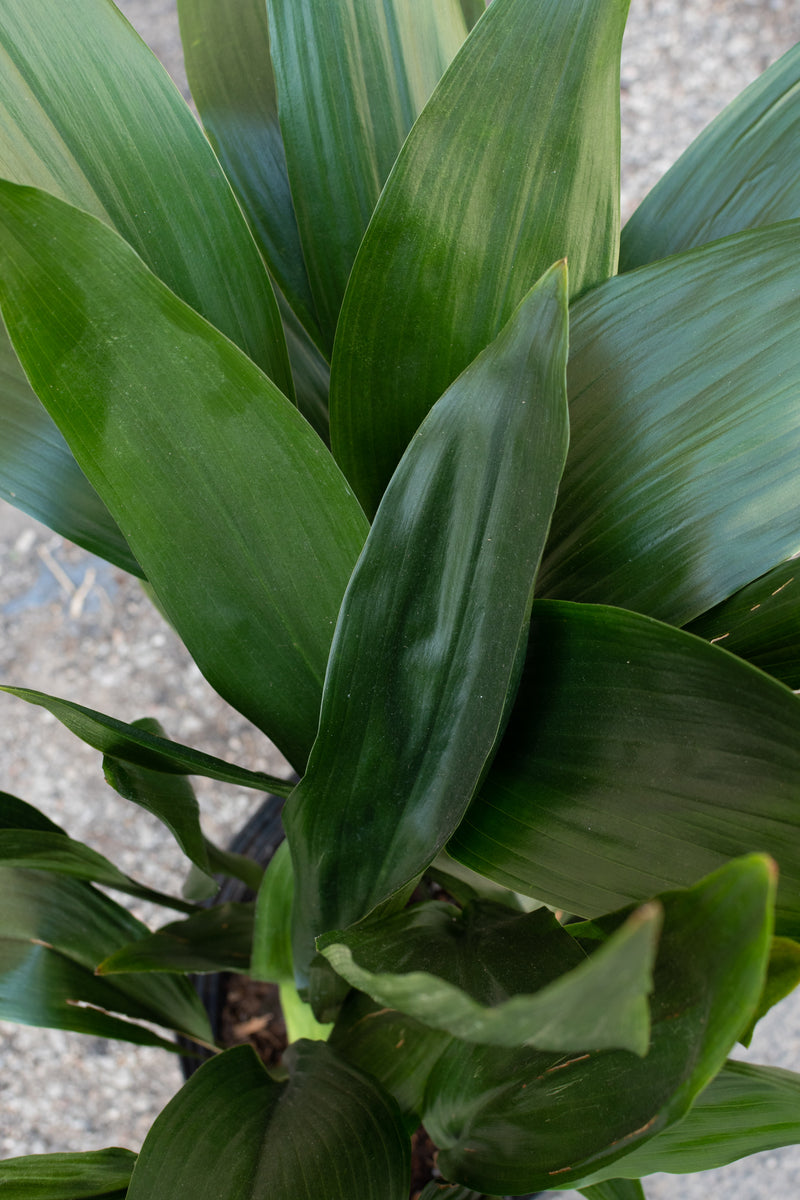The photo captures a vivid, top-down view of a lush, green potted plant with smooth, wide, blade-like leaves, varying in shades of green. The leaves predominantly appear flat from this angle, with their surfaces glistening in the sunlight. Some leaves show subtle, thin variegation with lighter and darker green stripes. There are visible signs of slight wear, such as some browning tips and small slices on a few leaves, likely due to normal wear and tear. The leaves are densely packed, obscuring most of the plant's body, while the black plastic rim of the pot and a bit of brown soil or planting chips peek through at the base. The background appears to depict an outdoor setting with a speckled, grayish surface, possibly asphalt or a dirt path with wood chips and dead grass. The overall scene conveys a healthy, thriving plant, accentuated by the sun-splattered, chlorophyll-rich leaves.